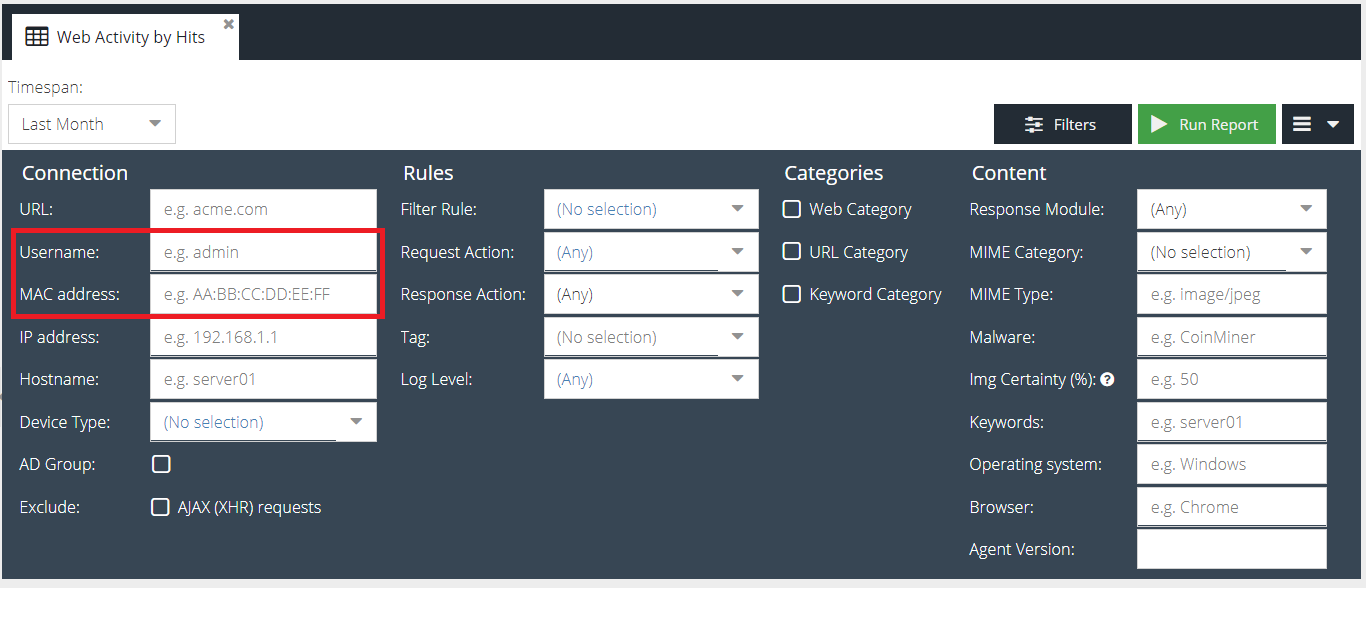Here's the cleaned-up and detailed caption:

---

**Screenshot of Web Activity Panel:**

The screenshot presents a detailed web activity panel that captures various elements of an analysis dashboard. The primary screen is a combination of a calendar/chart on the left side and multiple data filters, options, and metrics on the right.

Key headings and sections include:

- **Time Span:** Options for selecting the period of activity being analyzed, such as "Last Month."
- **Filters:** Tools to refine data views.
- **Run Script:** A functional button for executing custom scripts.
- **Hamburger Icon:** An icon presumably leading to additional settings or a menu.

### Connection Section:
- **URL**
- **Username:** Surrounded by a red rectangle.
- **MAC Address:** Also highlighted with a red rectangle.
- **IP Address**
- **Host Name**
- **Device Type**
- **AD Group**: Written as "Ad Group."

### Rules Section:
- **Filter Rule**
- **Request Action**
- **Response Action**
- **Tag**
- **Log Level**

### Categories Section:
- **Web Category**
- **URL Category**
- **Keyword Category**

### Content Section:
- **Response Module**
- **MME Category**
  - **MME Type:** Specified as "Malware."
  - **Image Certainty (IMG):** Followed by a percentage sign and a question mark in parentheses.
- **Keywords**
- **Operating System**
- **Browse**
- **Agent Version**

The comprehensive layout and detailed categorization support in-depth analysis of web activity, providing significant insight into connections, rules, content, and various categories essential for web monitoring and security assessment.